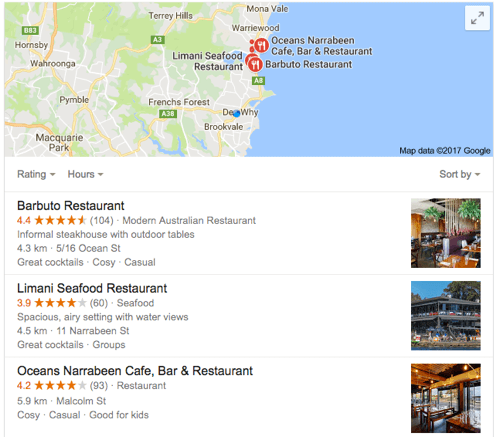The image depicts a Google Maps interface focusing on the coastal area of Australia. Several red markers are scattered across the map, indicating the locations of various restaurants in the highlighted region. Below the map, there is a detailed chart presenting an organized list of these restaurants. 

The chart's header includes categories such as 'Ratings,' 'Hours,' and a 'Sort By' option situated on the far right. The list begins with Barbuto Restaurant, which boasts a rating of 4.4 stars based on 104 reviews. This establishment offers modern Australian cuisine and includes detailed information such as its address, notable features, and a photograph of its stylish interior.

Next on the list is Limani Seafood, rated 3.9 stars from 60 reviews. Known for its seafood offerings, the entry also features an exterior image of the restaurant building.

The third restaurant noted is Ocean Nairobene Cafe, Bar, and Restaurant, which holds a 4.2-star rating from 93 reviewers. This listing is accompanied by an image of its indoor seating area.

The chart is designed with a white background and black text, while the star ratings and accompanying star icons are highlighted in orange, making it visually easy to evaluate and compare the options.